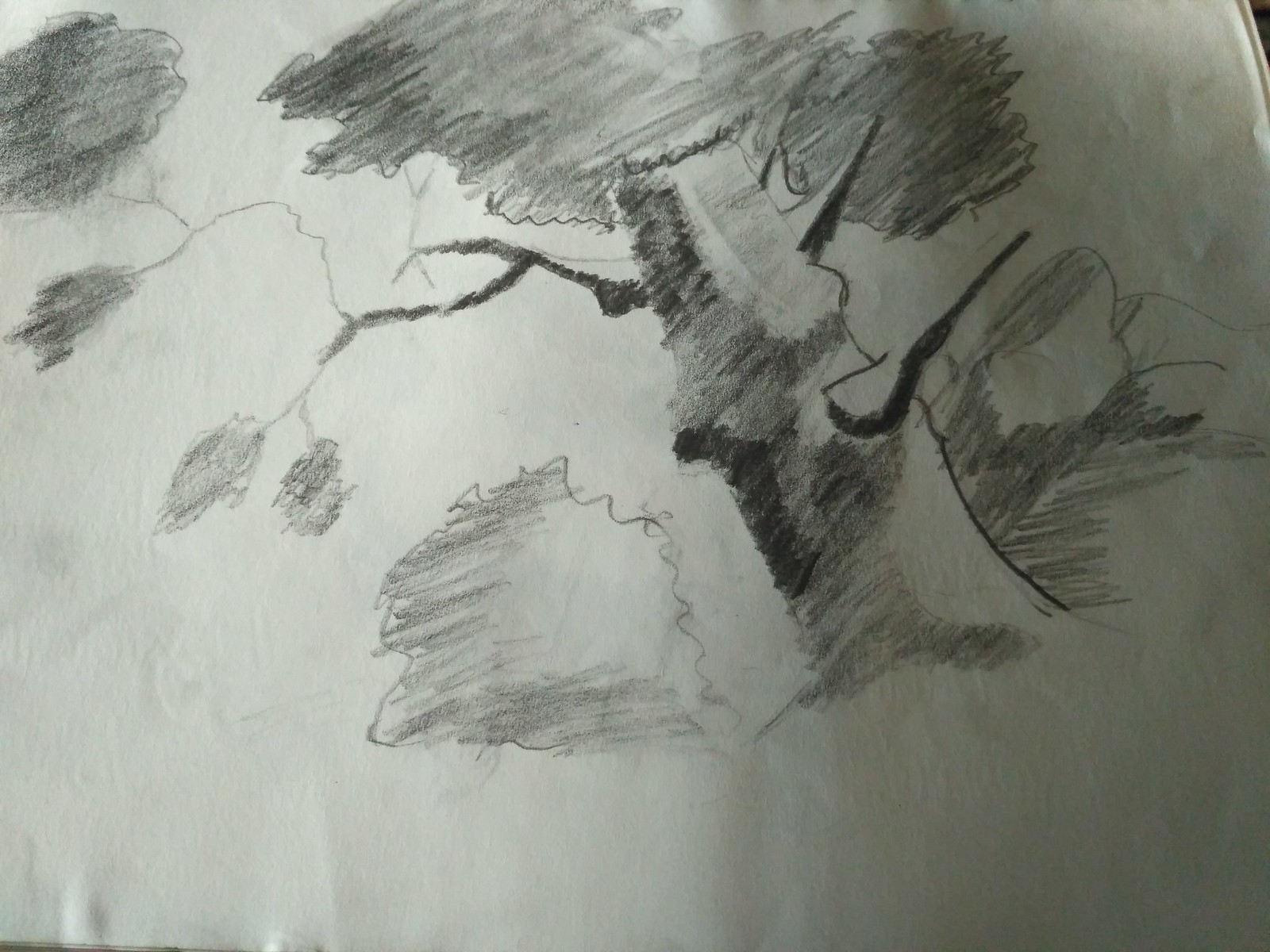This pencil-shaded drawing, reminiscent of charcoal artistry, is presented on a slightly crinkled piece of white paper, with noticeable creases in the upper right and bottom left corners. The central subject is a tree, flanked by bushes on both sides. The bushes, depicted through meticulously applied gray shading, frame the composition. The tree's wide trunk is rendered with a gradient of shading, transitioning from a lighter right side to a progressively darker left side, culminating in the deepest shadows on the far left. About halfway up the trunk, an empty branch juts out to the right. Further up, near the two-thirds mark of the tree's height, a larger branch extends horizontally, with the left end branching off into a splintered segment adorned with darkly shaded leaves. The foliage at the tree's apex is densely shaded, adding depth and contrast to the overall scene.